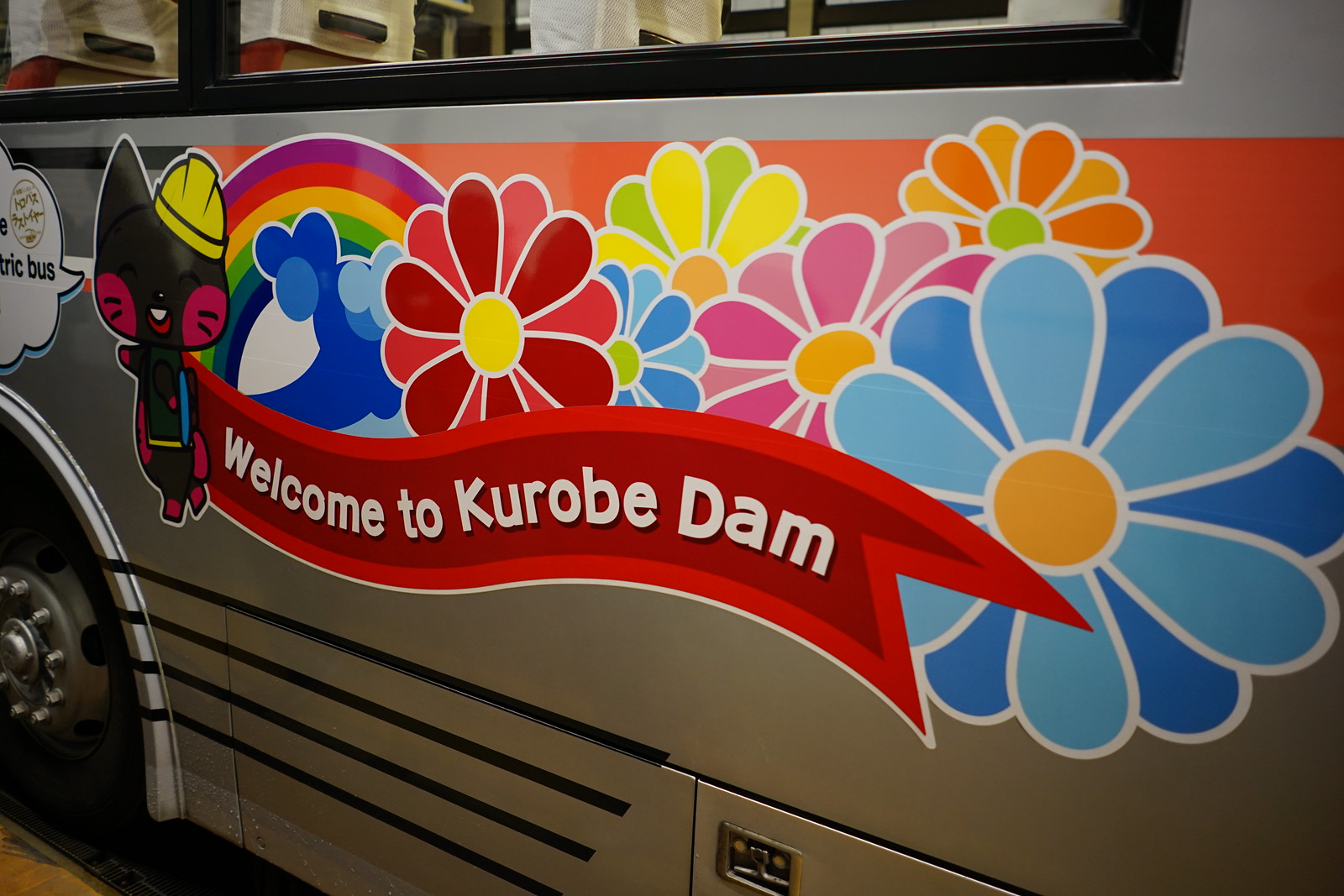This photograph captures the side of a vibrant gray bus with black trim and windows framed in black. The focal point of the artwork is a colorful, hand-painted design featuring a large rainbow on the left side, followed by an array of beautifully detailed flowers in various bright hues—blue, pink, orange, yellow, and red—with centers in shades of yellow and orange. The flowers are intricately painted, showcasing various combinations of petals: a two-toned red flower with a yellow center, a smaller blue flower with a green center, a yellow and green flower with an orange center, and a prominent blue flower with a gold center. Among these colorful details is an adorable, fictional creature standing on one end of the bus. This character, with a comical appearance, wears a hat and earmuffs and is dressed in a cute outfit that includes pink shoes and a yellow belt. The creature stands next to a banner that reads "Welcome to Korobe Dam," written in white letters on a red ribbon outlined in a lighter red hue. Above this lively artwork, the bus windows are slightly visible, and below, the shiny black wheels with silver rims are partly seen. The overall effect of the painting, combined with the natural elements of the bus, creates an inviting and whimsical scene.